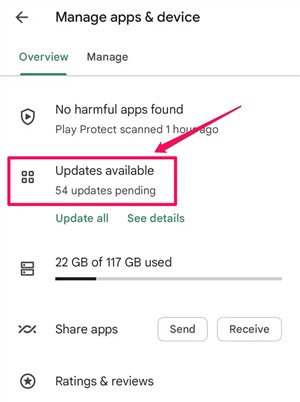A cell phone screenshot displays a section labeled "Manage Apps & Device." An arrow points to the left of this section, and beneath it, "Overview" is highlighted in green with a green line underneath. Next to "Overview," the word "Manage" appears in black text. A faint gray line separates this area from the next section, which features a shield icon and the message "No harmful apps found." Below, in smaller print, it reads "Play Protect, scanned 1 hour ago."

A prominent red border encircles the "Updates available" section, indicating 54 updates pending. Adjacent to this, four circles are aligned—two at the top and two at the bottom. A red arrow points downward toward the updates section. Below this area, green buttons for "Update all" and "See details" are visible.

Further down, storage information is displayed, showing "22 GB of 117 GB used." The screen also features options for "Share apps" with "Send" and "Receive" buttons nearby. The section concludes with "Ratings and reviews" accompanied by a star icon.